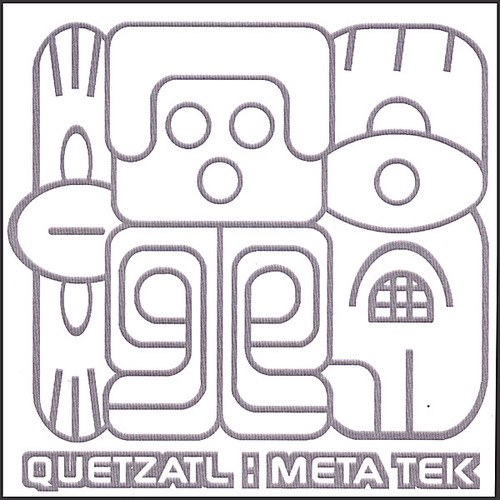This image depicts a stylized male character with a distinct, blocky appearance. His head is represented by a square with three circles, presumably illustrating his eyes and mouth. His hair is rendered in a chunky, angular fashion. The character's body is another square-like shape featuring inward swirls, likely symbolizing his arms and legs.

To his left, there's an oblong disc shape featuring several ovals cut out, resembling a sideways eye mask. On the right side of the image, there are two rectangular shapes positioned at the bottom. The caption "Quetzal Metatepe" is inscribed below the illustration.